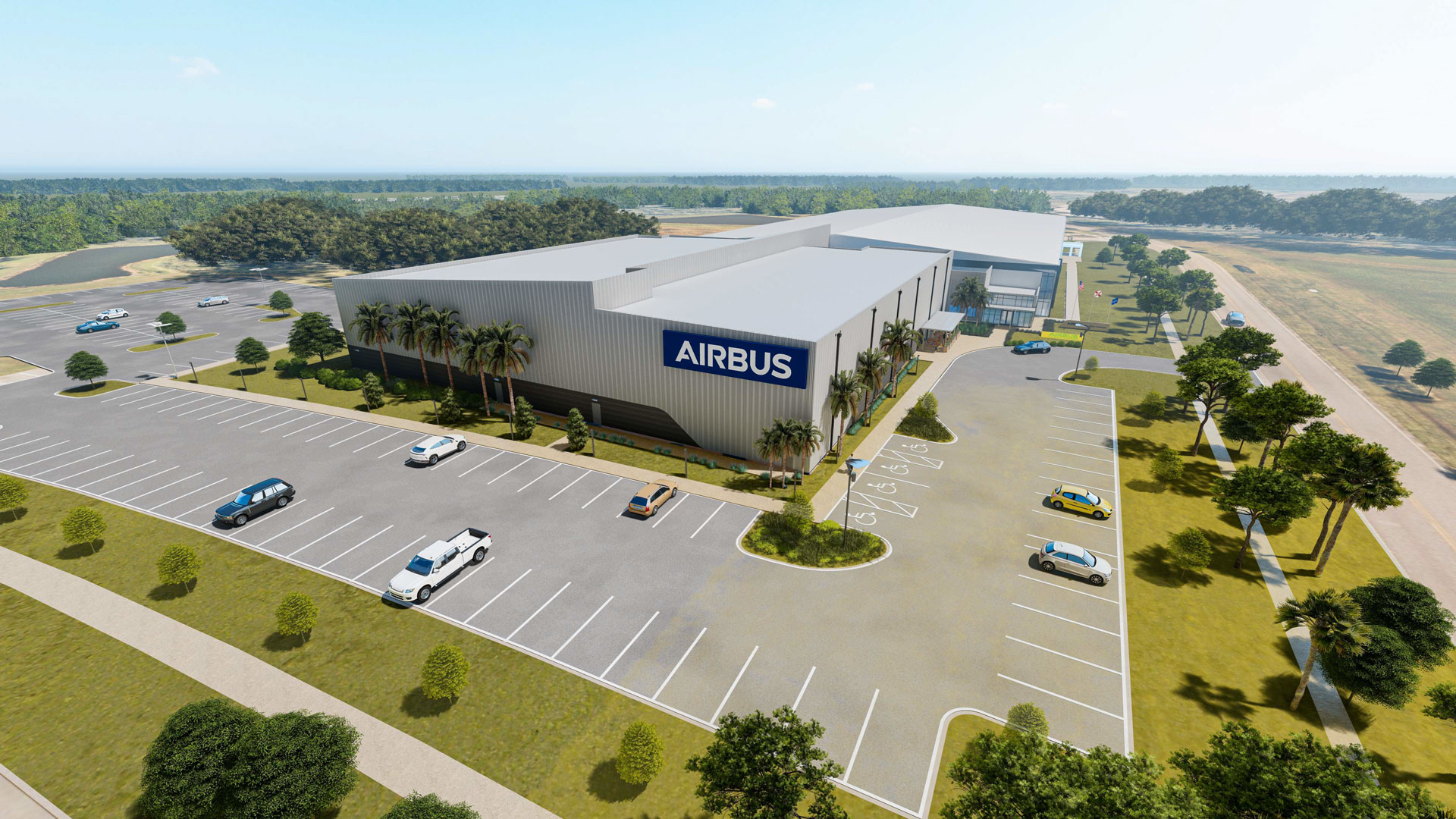The image is an aerial photograph of an industrial-style office building bearing the name "Airbus." The building has a prominent blue sign with white lettering and a white metal exterior with a white roof. The photograph captures a large parking lot surrounding the building, with a variety of cars that may appear somewhat artificial, indicating the image could be a 3D render. The lot is mostly empty, showing sparse cars such as a black, a tan, several blue, and multiple white ones, with some cars possibly not parked in designated spots. Handicapped parking spots are visible, painted white, towards the middle of the image.

The scene is detailed with landscaping, including tall palm trees, shorter shrubs, and green grass. There are sidewalks around the building, with additional fields and greenery on the right side of the image. In the background, a blue sky extends across the top of the photo, transitioning to a whiter hue towards the right, with tall green trees spanning the horizon. There appears to be a blue and white building with a white roof situated behind the main Airbus building. Additionally, there is a roadway running along the right side of the property. The perspective suggests that the image might be taken from a higher vantage point, such as a neighboring tall building or a low-flying helicopter.